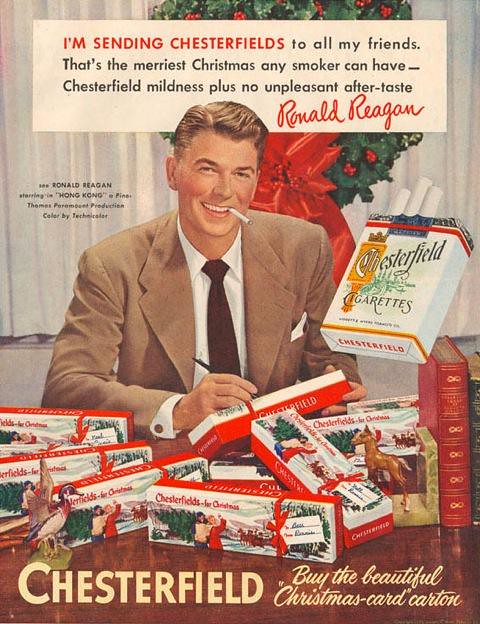This vintage magazine advertisement for Chesterfield Cigarettes features Ronald Reagan, who was a prominent movie star at the time and later became President of the United States. The ad is Christmas-themed, with a festive backdrop including a large wreath adorned with a big red ribbon. At the top of the image, a white banner overlapping the wreath reads, "I'm sending Chesterfields to all my friends. That's the merriest Christmas any smoker can have. Chesterfield mildness plus no unpleasant aftertaste," and is signed by Ronald Reagan. 

Ronald Reagan, depicted in a brown suit and black tie, is shown sitting at a desk with a pile of Chesterfield cigarette cartons that have a special Christmas design with a "To and From" section, suggesting they are intended as gifts. Reagan, with a cigarette in his mouth, appears to be signing or addressing the cartons. To the right, an oversized pack of Chesterfield cigarettes is prominently displayed. The advertisement includes the Chesterfield logo at the bottom left and the catchphrase, "Buy the beautiful Christmas card carton," in light beige-orange cursive at the bottom right. The image, which seems to be hand-drawn in a realistic manner, captures the holiday spirit and emphasizes the mildness and lack of unpleasant aftertaste of Chesterfield cigarettes.